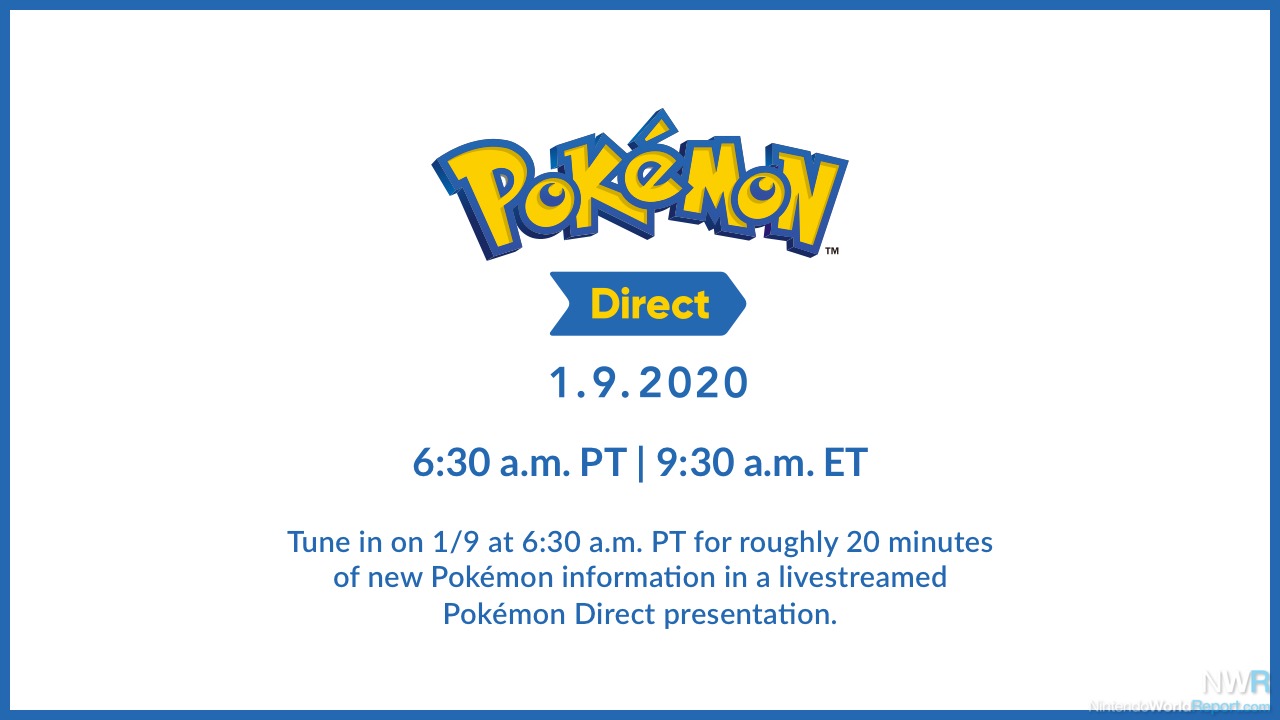A promotional advertisement for a Pokémon event set against a predominantly blue and white color scheme. The ad features a large, blue-outlined square banner with the iconic Pokémon logo prominently displayed at the center. The logo, in its traditional yellow color with blue outlining, is accompanied by a trademark symbol.

Below the logo, a blue banner with yellow text reads "Pokémon Direct." The specifics of the event are clearly detailed: the date "1.9.2020" is in a matching blue hue, with times listed as "6:30 a.m. PT" and "9:30 a.m. ET." 

The advertisement encourages viewers to "Tune in on 1.9 at 6:30 a.m. Pacific Time for roughly 20 minutes of new Pokémon information in a live stream Pokémon Direct presentation." Despite lacking a web address or additional navigation details, the minimalist design effectively conveys the necessary information, utilizing up to four distinct font styles for emphasis and clarity. The overall visual feels reminiscent of the size and structure of a business card, enveloped in consistent blue and yellow tones.